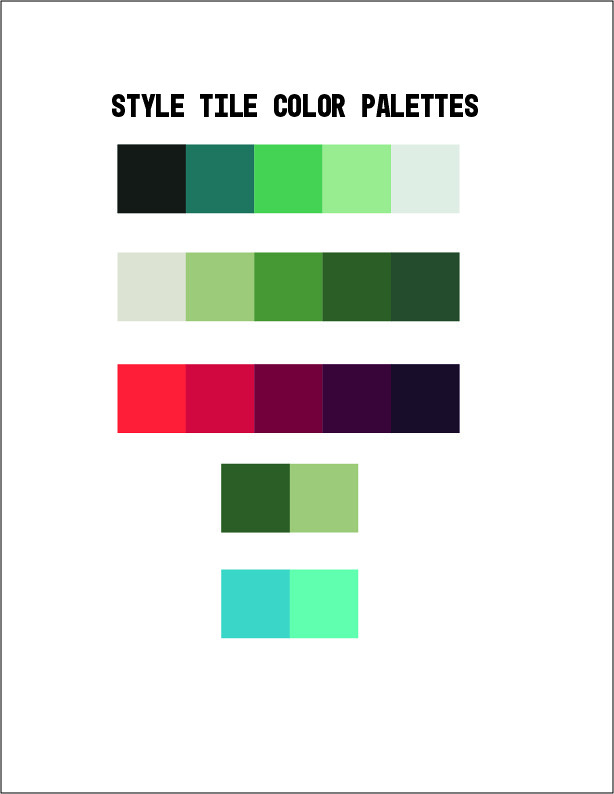The image features a white background with black text in all capital letters at the top that reads "STYLE TILE COLOR PALETTES." Below the text, there are five distinct rows of rectangular shapes, each composed of color blocks. The top row consists of a horizontal rectangle made up of five adjacent squares, with colors transitioning from black to dark green, medium green, lighter green, and finally to a very light gray with a hint of green. The second row is a similar rectangle of five squares starting with a grayish white, followed by pea green, medium green, dark green, and forest green. The third row contains a gradient of five squares progressing from bright red to muted red, reddish pink, purplish pink, and ends in a black or very dark purple. The fourth row features two squares in a horizontal rectangle transitioning from dark green to lighter green. The fifth and final row also comprises two squares, shifting from a turquoise or cyan green to a seafoam green. Each rectangular shape is bordered by a thin black line, unifying the color blocks against the white backdrop.